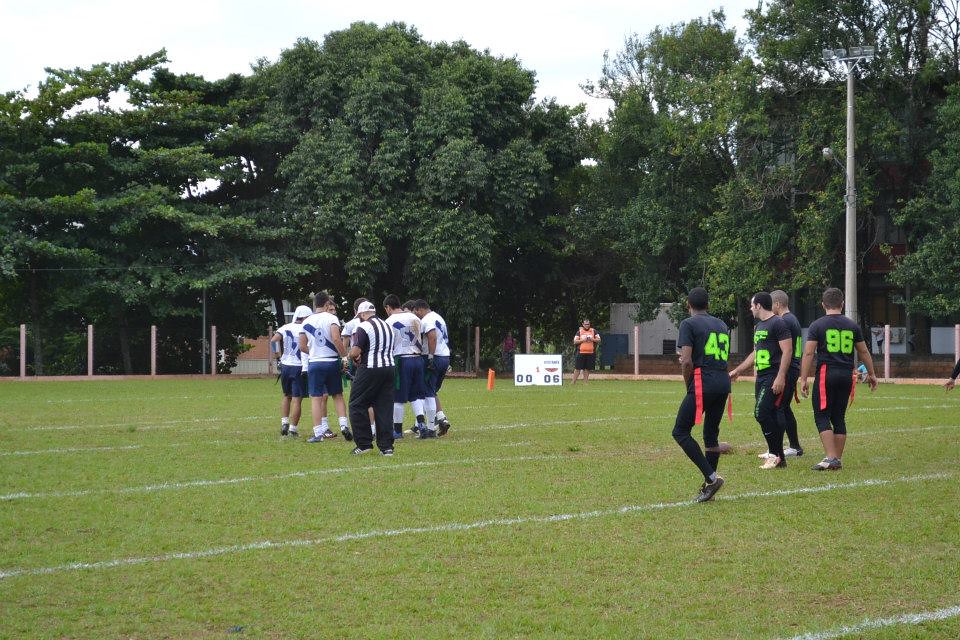In this daytime photograph of a flag football game, we see two teams on a lush green football field marked with white lines. On the right side of the image, a group of four players is huddled together, all wearing black uniforms with neon green numbers on their backs, paired with black pants, and equipped with red flags on their hips. To the left, another team is in white jerseys with a blue diagonal stripe and matching blue shorts. This team has green flags on their hips. A referee, easily identifiable in a striped shirt and black pants, stands near the white team's huddle. In the background, a row of large trees creates a natural barrier, partially concealing various structures. Also visible near the center of the photo is a small scoreboard attended by a person in an orange vest. Additional individuals, including one walking a bicycle, appear to be in the vicinity of the field, suggesting casual observers rather than a formal audience.